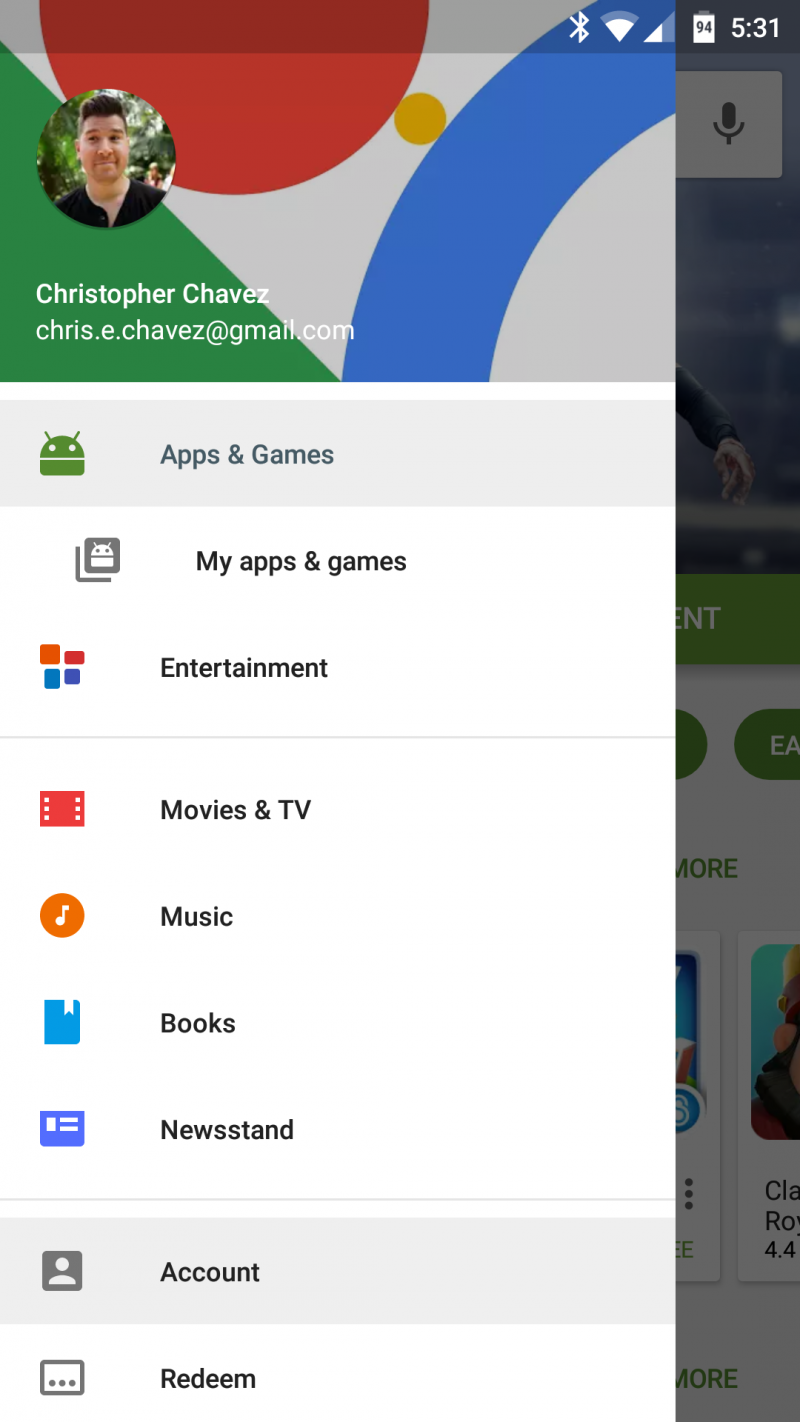The image is a screenshot taken from someone's phone, displaying a menu with various options. At the top left, there's a circular profile picture of a man, identified as Christopher Chavez with the email address chris.e.chavez@gmail.com displayed below the name. The background behind him consists of geometric shapes: a partially visible red circle at the top, a green triangle on the left, a yellow circle in the center, and a blue curved segment on the right.

The timestamp on the phone shows 5:31, and the battery is 94% charged. The right side of the screenshot features a semi-transparent gray overlay with various clickable icons faintly visible.

The main menu on the left, beneath Christopher Chavez's profile information, includes several categories with corresponding icons: "Apps and Games," "My Apps and Games," "Entertainment," "Movies and TV," "Music," "Books," "Newsstand," "Account," and "Redeem." These options populate the left column, organized vertically with their respective text labels and icons.